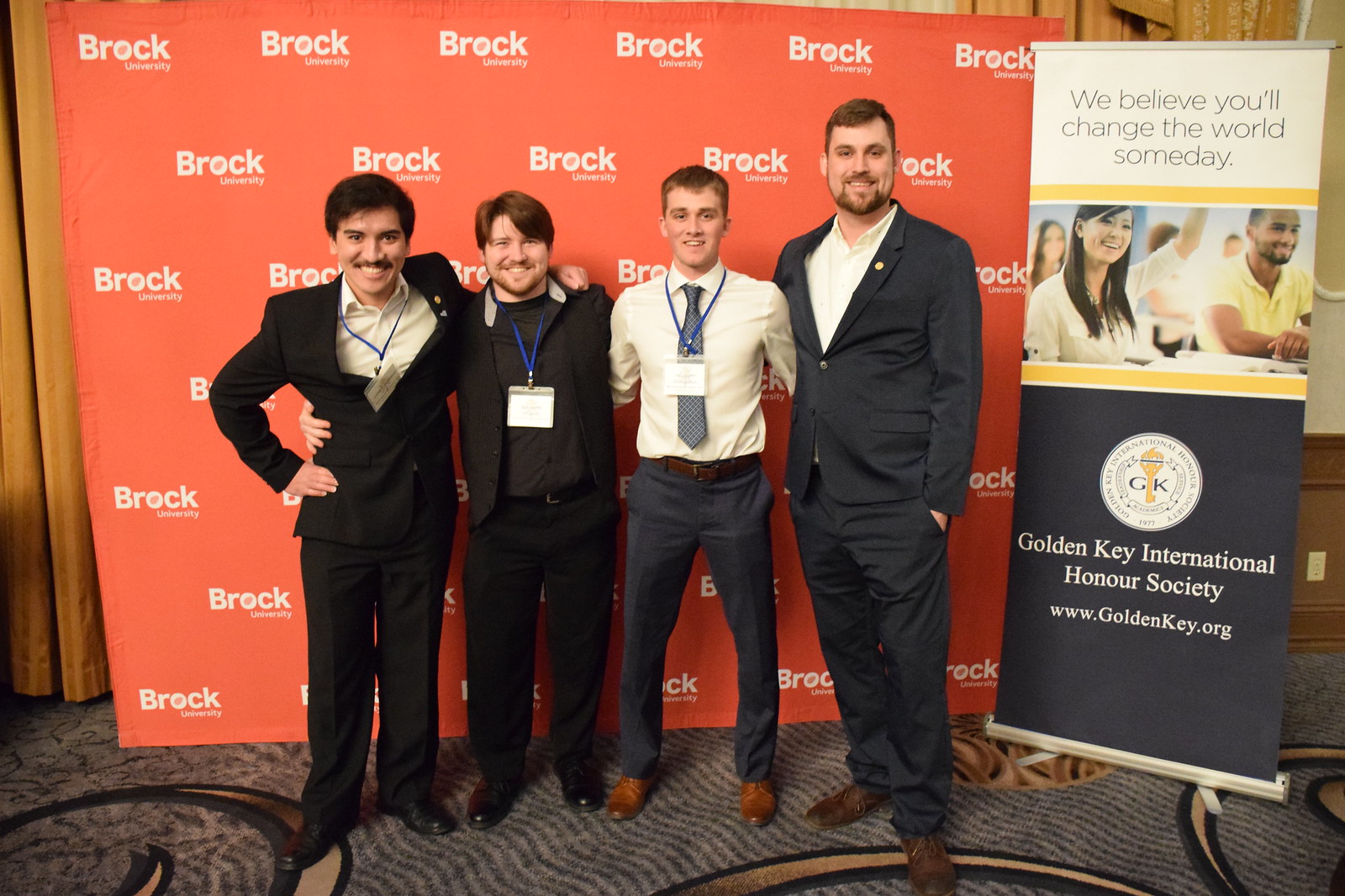The photograph showcases four men standing in front of an orange step-and-repeat banner emblazoned with the white "Brock University" logo. From left to right, the first man is dressed in a dark suit with a white shirt and a lanyard around his neck. He has dark hair and a mustache. The second man, slightly shorter, also wears a dark suit and a dark shirt, complete with a lanyard. He sports brown hair and a brown beard and mustache. The third man, slightly taller than the second, is dressed differently, wearing blue slacks, a brown belt, a white button-up shirt, and a tie, along with a lanyard. He has light-colored short hair. The fourth man, the tallest, is in a dark suit with a white shirt and features a lapel pin. He, too, has a brown beard and brown hair. They are all smiling, with their arms around each other's shoulders or waists, exuding a sense of camaraderie.

To their right, a sign reads, "We believe you'll change the world someday. Golden Key International Honor Society" alongside a URL, www.goldenkey.org. They stand on a carpet featuring swirly designs, further framing the scene with a cohesive aesthetic.